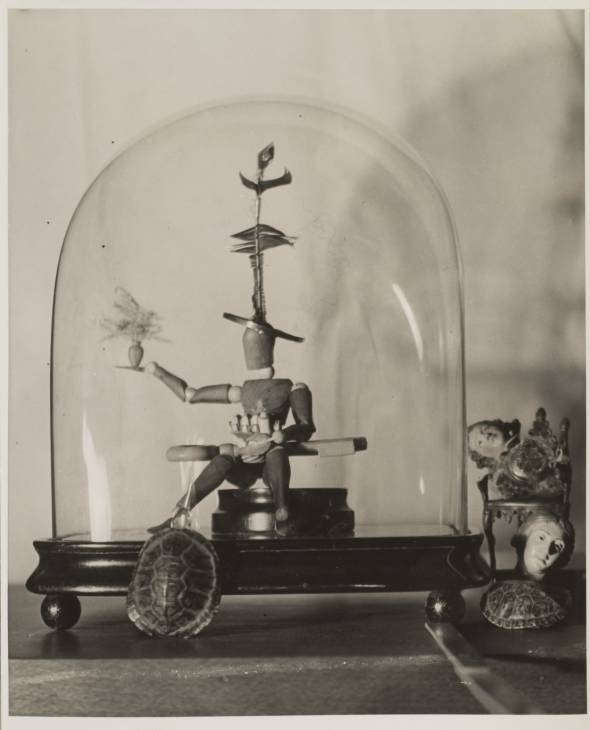The black and white photograph captures a carefully staged curio display within a glass enclosure, which sits atop a dark wooden base. At the center of the image is an articulated anatomical model or figurine, posed sitting on a pedestal inside the enclosure. The figurine sports a whimsical hat characterized by a wide brim and a tall, column-like ornament protruding from the top, giving it a playful appearance. Its right hand extends to hold a flower pot or vase filled with small flowers. Outside the glass enclosure, a tortoise shell leans against the base, adding an organic touch to the vignette. To the right of the display case, there are porcelain figures or doll heads, one of which is positioned on a small chair, contributing to the eclectic and slightly surreal composition.